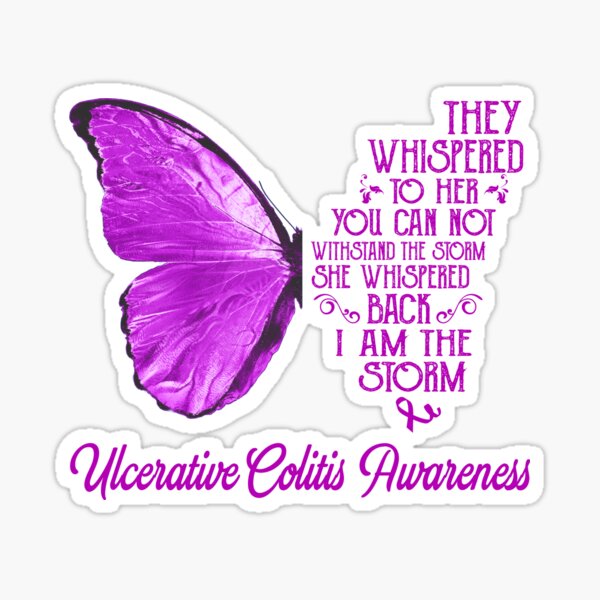The image features a detailed digital drawing with a gray background. Dominating the left side is a purple butterfly rendered in a side view, encased in a thin gray outline. The butterfly's delicate wings extend toward the top left and bottom right corners of the image, adding an elegant touch.

Adjacent to the butterfly on the right side, there is a poetic and inspirational quote, positioned inside a light blue bordered area. The quote, in purple letters, reads:

"THEY WHISPERED TO HER,  
'YOU CANNOT WITHSTAND THE STORM.'  
SHE WHISPERED BACK,  
'I AM THE STORM.'"

Adorned with small swirl designs beside the word "back" and floral motifs near "to her" and below "storm," these embellishments enhance the visual appeal. Below the quote, another gray-bordered section contains the phrase in purple letters:

"ULCERATIVE COLITIS AWARENESS"

The composition harmoniously combines art and text to deliver a strong message of resilience and awareness.